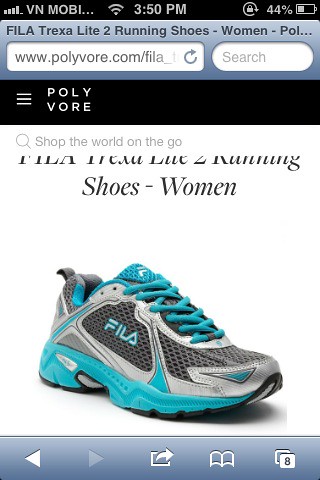The screenshot appears to be taken from an older cell phone, characterized by a more compact and less elaborate display. At the top of the screen, a black bar shows various indicators: four bars of service, the carrier name 'VN Mobi', a Wi-Fi symbol, the time '3.50 PM', an additional symbol, and the battery status at 44% with a visual battery indicator. Below this, a search field features the gray placeholder text "Fila Trexa Lite 2 Running Shoes - Women," above a URL input showing "www.polyvore.com/fila_." There's an empty search box to the right of this URL field. The website displayed on the screen is Polyvore. The interface includes a black bar featuring a drop-down menu on the left and the white text “Polyvore” to the right. Below, the product name "Fila Trexa Lite 2 Running Shoes - Women" is written in black font, accompanied by an image of a running shoe. The shoe is predominantly gray with dark blue soles and teal laces, marked with the brand name 'Fila'. Additional symbols and a number '8' appear at the bottom right corner of the image.